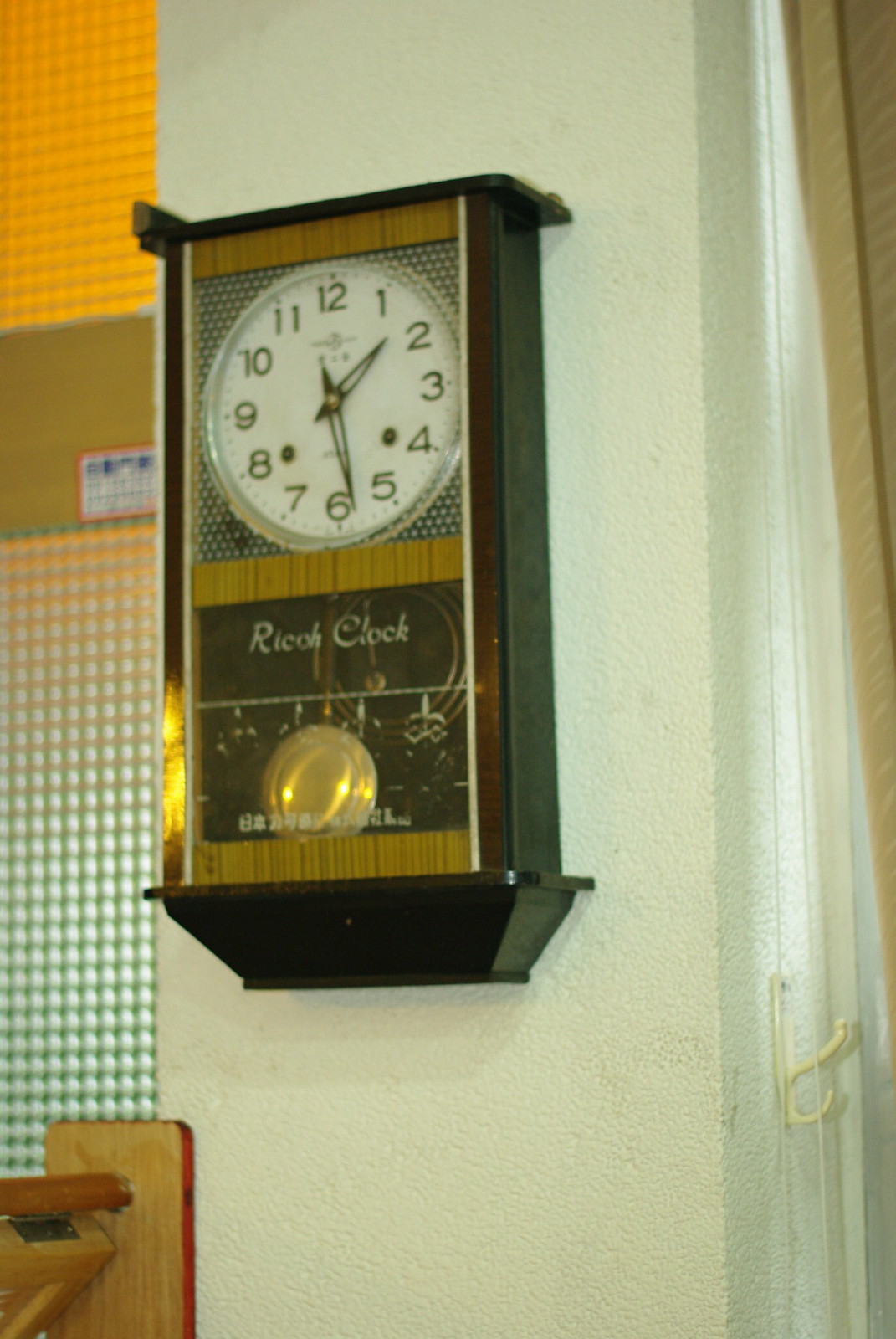The image captures an indoor scene primarily focusing on an old-fashioned wall clock mounted at the center of a wall that is a bright white, albeit slightly chipping at the corners. The clock, framed in dark brown wood with a light brown interior, is rectangular in shape with its lower portion forming a rhombus. The background of the clock features a polka-dotted pattern in black and white. The dial of the clock displays numbers 1 through 12, with the time set at almost 1:29. Below the clock face, a gold pendulum swings back and forth, and the name "Rico Clock" is printed in gold lettering above it. To the right of the image, a small white plastic hook is attached to the wall next to light brown curtains adorned with a subtle pattern, which extend from the upper to the bottom right corner. Additionally, a textured beige wallpaper is visible on the left side of the clock, alongside a frosted glass area with circular patterns obstructing the view.